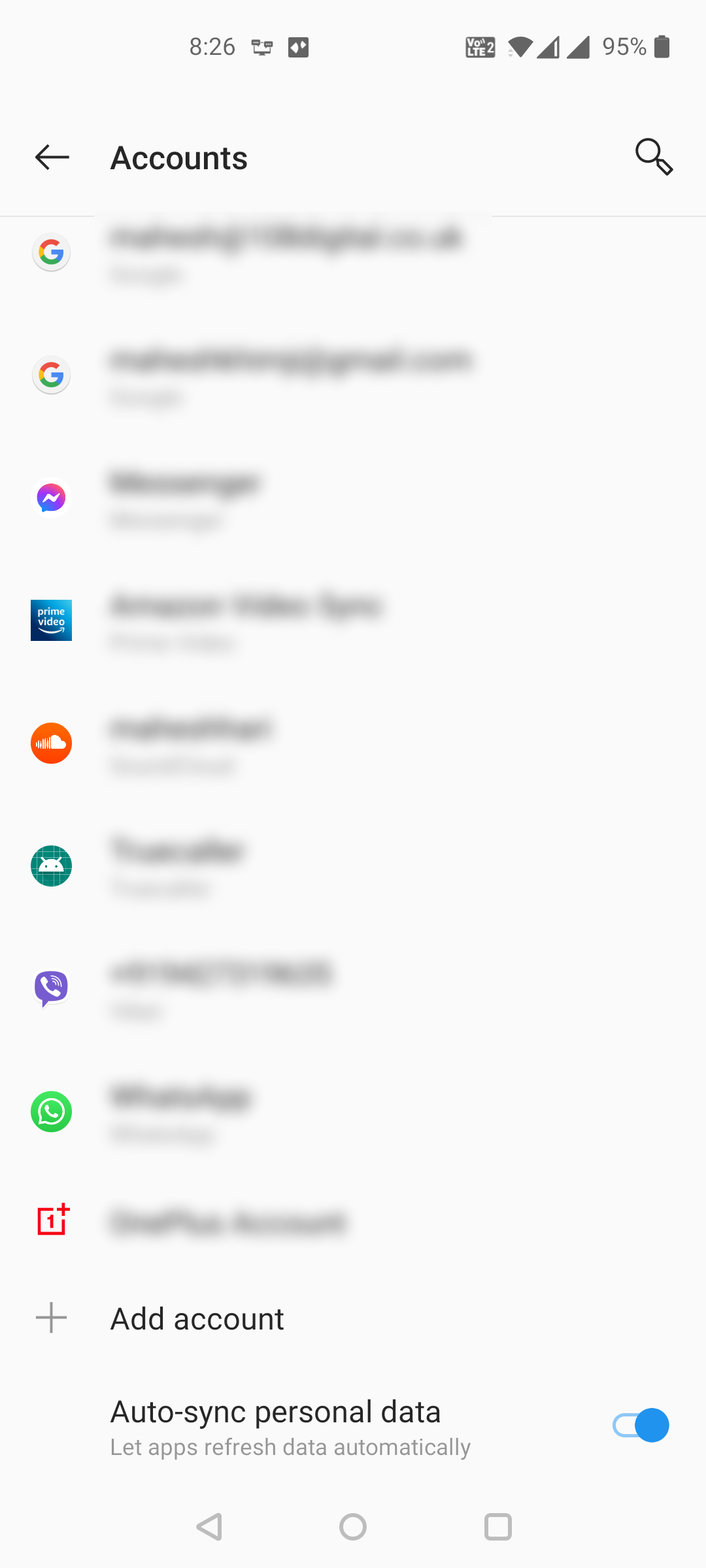A screenshot displays various smartphone interface elements in a blurry manner. At the top of the screen, the Wi-Fi signal strength shows 94%. Below this, there are several icons and symbols, most of which are not clear due to the blurriness. Among the visible symbols are a left arrow, a magnifying glass, a 'G', and several squares and circles in orange and blue, indicating different apps or settings. The primary content of the screen appears to be a settings menu with an option to toggle "Auto-dashing personal data," allowing apps to refresh data automatically. The background is white, with different icons and text being blurred, suggesting the screenshot is meant to show account settings or app management on a smartphone.